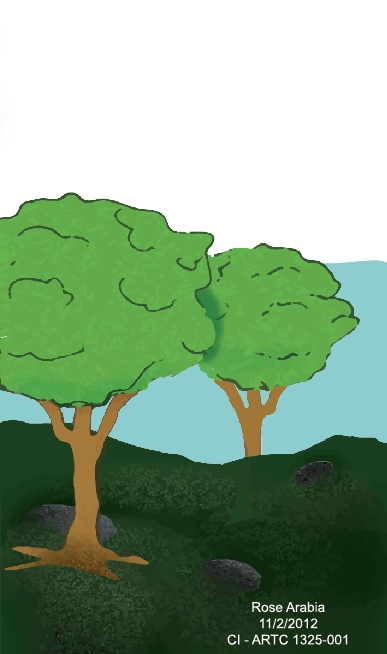This digitally created image features two nearly identical trees situated in a hilly green terrain. Both trees possess light tan trunks and leafy tops that resemble balls of lettuce in a light green hue. The tree in the background, while similar, appears partially obscured as its trunk is cut off by the sloping hill. Meanwhile, the tree in the foreground, positioned on the left-hand side, has its roots visibly embedded into the ground. Scattered around the terrain are various rocks, roughly the size of footballs or soccer balls, adding texture to the landscape. The sky transitions from a blue at the horizon to a white area above, through which the tops of the trees extend. At the bottom of the image, there is text that reads, "Rose, Arabia 11-2-2012 CI-ARTC 1325-001."